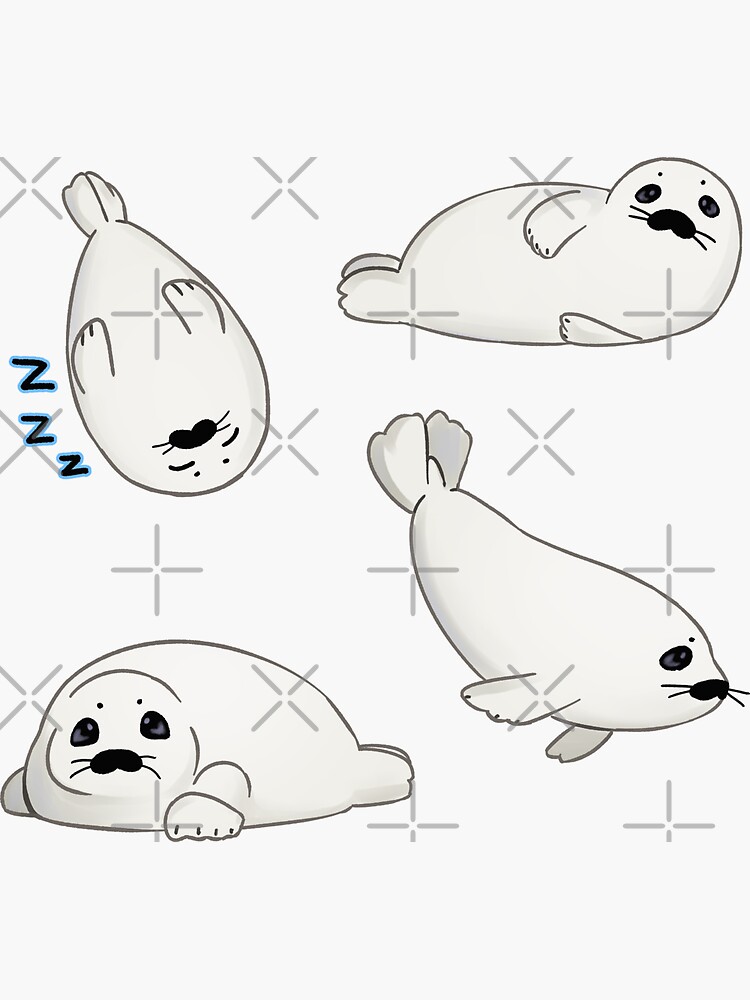The image is a detailed digital drawing of a white and black seal depicted in four different positions on a white background. In the top-left corner, the seal is upside down, facing the viewer with bead-like eyes, a nose with whiskers, and little flippers resting on its body. Beside it, to the right, another seal is laying on its back with its belly exposed, head turned towards us, rounded eyes with spots above them, and three black Z's with a blue border indicating it is asleep. Its left flipper rests on the ground while the right is across its belly, and its feet are pointed outwards. On the bottom-left side of the drawing, a seal is shown laying on its stomach at an angle, facing the viewer. The final seal, located on the bottom-right, appears to be swimming; its tail is upwards and to the left, with its nose down and to the right, and its flippers are thrust back. Watermarks in the form of gray X’s and crosses are scattered throughout the background to prevent unauthorized use.